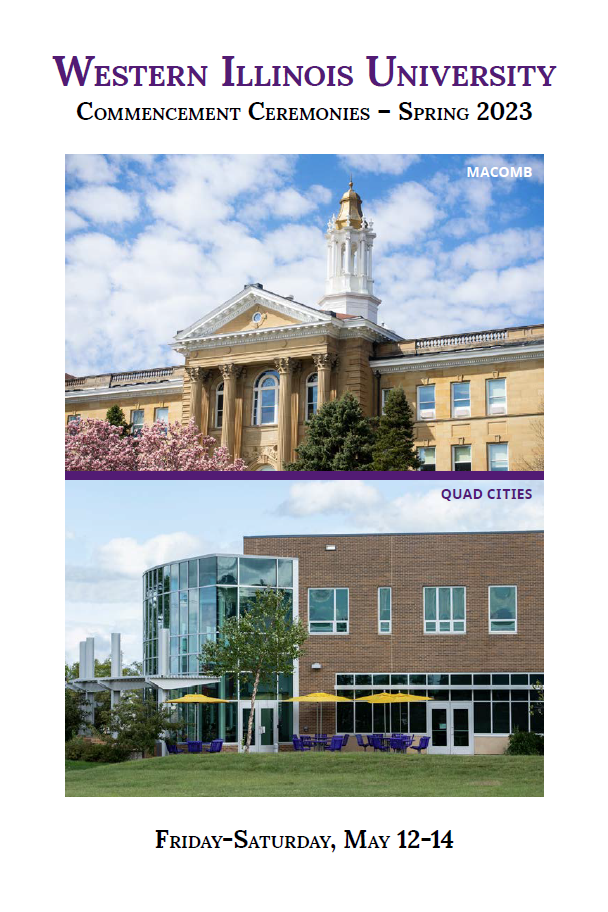The image is a promotional poster for the "Western Illinois University Commencement Ceremonies, Spring 2023" and features elegant serif font in a subtle shade that appears purple or black. Beneath the heading, there are two distinct photographs, representing different university campuses.

The top image labeled "Macomb" showcases a stately, historic building crafted from tan brick. Notable architectural elements include classic columns at the entrance and a prominent cupola, which may be a carillon, crowning the structure.

The bottom image labeled "Quad Cities" depicts a contemporary building characterized by brown brick and features at least a two-story glass atrium that enhances the entryway.

The poster concludes with the event dates, listed as "Friday through Saturday, May 12th through 14th," inviting graduates and their families to the ceremonies.